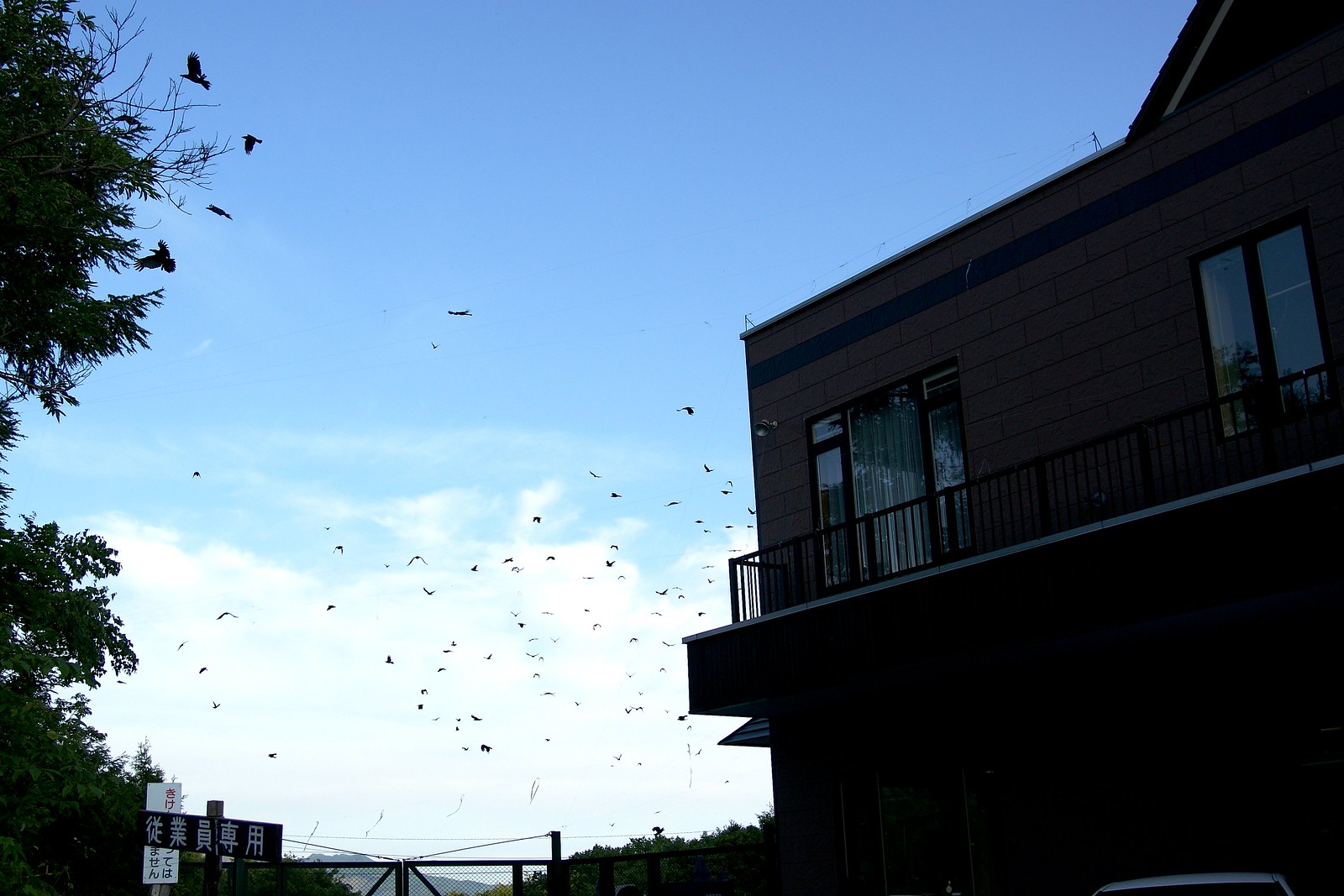This photograph captures a two-story building from a ground-up perspective, prominently occupying the right side of the image. The building, with its dark brown façade, features large, tall glass windows on the second story and an adjoining little deck or continuous railing. The roof appears flat on one side before sloping upward. The bottom section of the building is minimally lit, revealing no distinct features. 

To the left of the building, the sky is mostly a clear, vibrant blue with scattered, fluffy white clouds. Silhouetted against this blue expanse are numerous birds, flying in various directions individually rather than as a cohesive flock. 

In the left foreground, we see tree branches and leaves extending into the frame. Further in the background on the lower left side, there is a dark-colored bridge and another brick building partially obscured by the distance. Additionally, the lower left corner of the photo contains two signs with Chinese characters, one with white text on a dark background and the other with dark text on a white background.